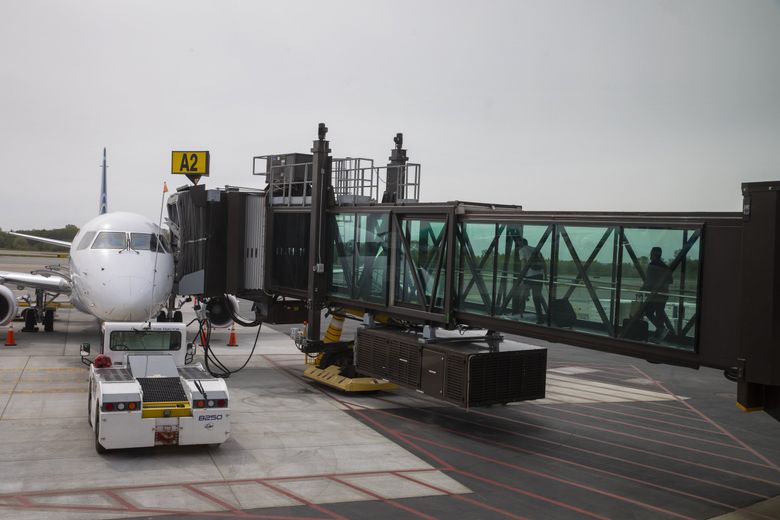The photograph captures a bustling airport scene on an overcast day, characterized by a lilac-blue sky. In the foreground, a mobile glass-covered boarding ramp allows passengers to board a small, white aircraft with a blue tail. The ramp’s structure includes many windows, some adorned with X marks, through which you can see at least two people pulling their suitcases. The ground beneath is a mix of gray and black, with distinct yellow stripes and red markers, indicating sections of the runway. A white vehicle, possibly a baggage transporter equipped with a conveyor belt, is parked facing the plane. Prominently displayed above the entry point to the plane is a yellow rectangular sign with black lettering that reads "A2." The photograph offers a detailed glimpse into the orderly process of aircraft boarding amidst a visually structured airport environment.